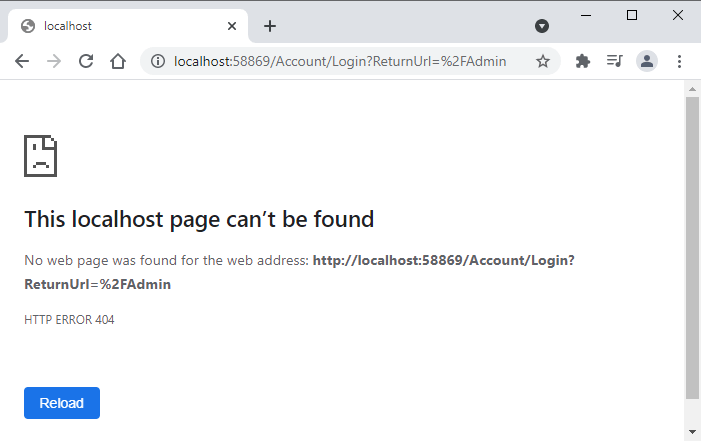A screenshot of a computer screen displays a web browser interface. At the top, a light gray horizontal bar spans the width of the screen, featuring a white tab labeled "localhost" in lowercase. To the left of this label is an icon, followed by a plus sign. On the far right of the gray bar are four symbols: a circle with a downward-pointing triangle, a dash, a square, and an X.

Beneath the gray bar, within the white tab area, there are navigation elements: a dark gray left arrow and a light gray right arrow, a circular arrow, a home button, an address bar for the web URL, and several other icons to the right.

Below this is a crisp white background divided by a faint gray horizontal line. This line separates the web browser's interface from the content area below.

The content area features a vertical rectangular box outlined in dark gray, illustrating a folded corner in the top right that obscures half of a sad face. The text beneath the sad face reads, in bold black font, "This localhost page can’t be found."

Further down, in black or gray font, it states, "No webpage was found for the web address," followed by the URL "http://localhost:58869/account/login?ReturnUrl=%2Fadmin" in bold.

The bottom of the error message reads "HTTP ERROR 404" in uppercase letters. To the left side of this message is a rectangular blue button with the word "Reload" in white.